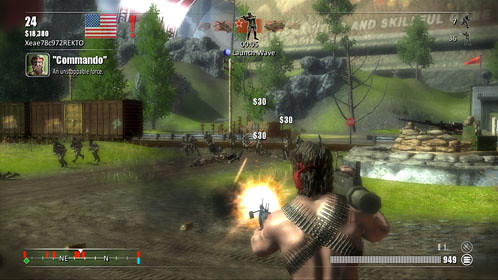In this intense in-game moment, a male character stands on a war-torn battlefield, viewed from behind. He has black hair and is equipped with a large missile launcher slung over his right shoulder. Ammunition belts are draped across his back, indicative of his heavy artillery role. In his left hand, he wields a machine gun that is actively firing, emitting bright light and vivid orange flames. The battlefield around him is chaotic, with dense smoke rising in the distance from numerous explosions. Amidst the grassy terrain, small soldier-like figures can be seen running, embodying the frantic pace and dynamic nature of this digital conflict.